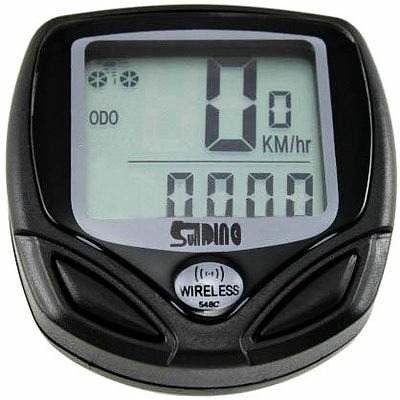An ultra-close image showcases a sleek, black measuring device, likely a stopwatch or fitness watch, against a pristine white background. The device is the sole focus of the frame, emphasizing its design and features. The rounded bottom and slightly curved sides frame the straight top, creating a streamlined silhouette. 

At the bottom corners are two elongated, triangular buttons, spaced apart, with a distinctive silver circular button labeled "wireless" positioned between them, slightly elevated. The digital display, encased in a silver border with a glass protective cover, dominates the upper portion of the device. 

In the upper-left corner of the display, two circular symbols are situated above the letters "ODO." Adjacent to the symbols, the display reads "0 KM/HR," suggesting a measurement in kilometers per hour. Below a dividing black line, four zeros indicate that no time has been set or recorded. This detailed composition underscores the device's functionality and minimalist design.